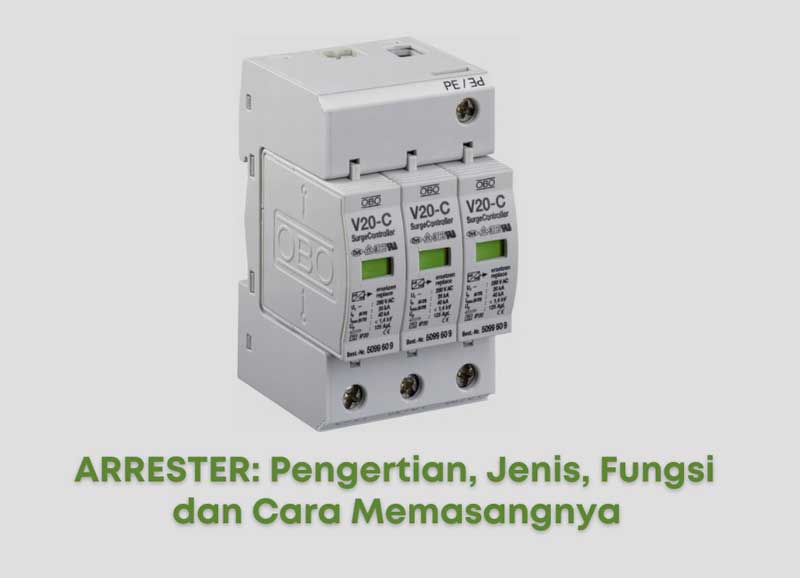The image depicts a vertical electrical device set against a light gray background, centrally positioned towards the top of the image with descriptive text below. The main object comprises three V20C surge controller fuses, each featuring a screw at the bottom and a window on the front. Notably, the top of the fuses is labeled PE, and the side of the device bears the letters OEO. The fuses and device body incorporate green elements within their design. At the bottom of the image, French text including "Arrester" is visible, along with other possibly non-standard terms like "Penjirtian," "Genus Fungsi," and "Dankara Memasangia," suggesting various functions or features. The overall presentation resembles that of a business slide or commercial product listing.